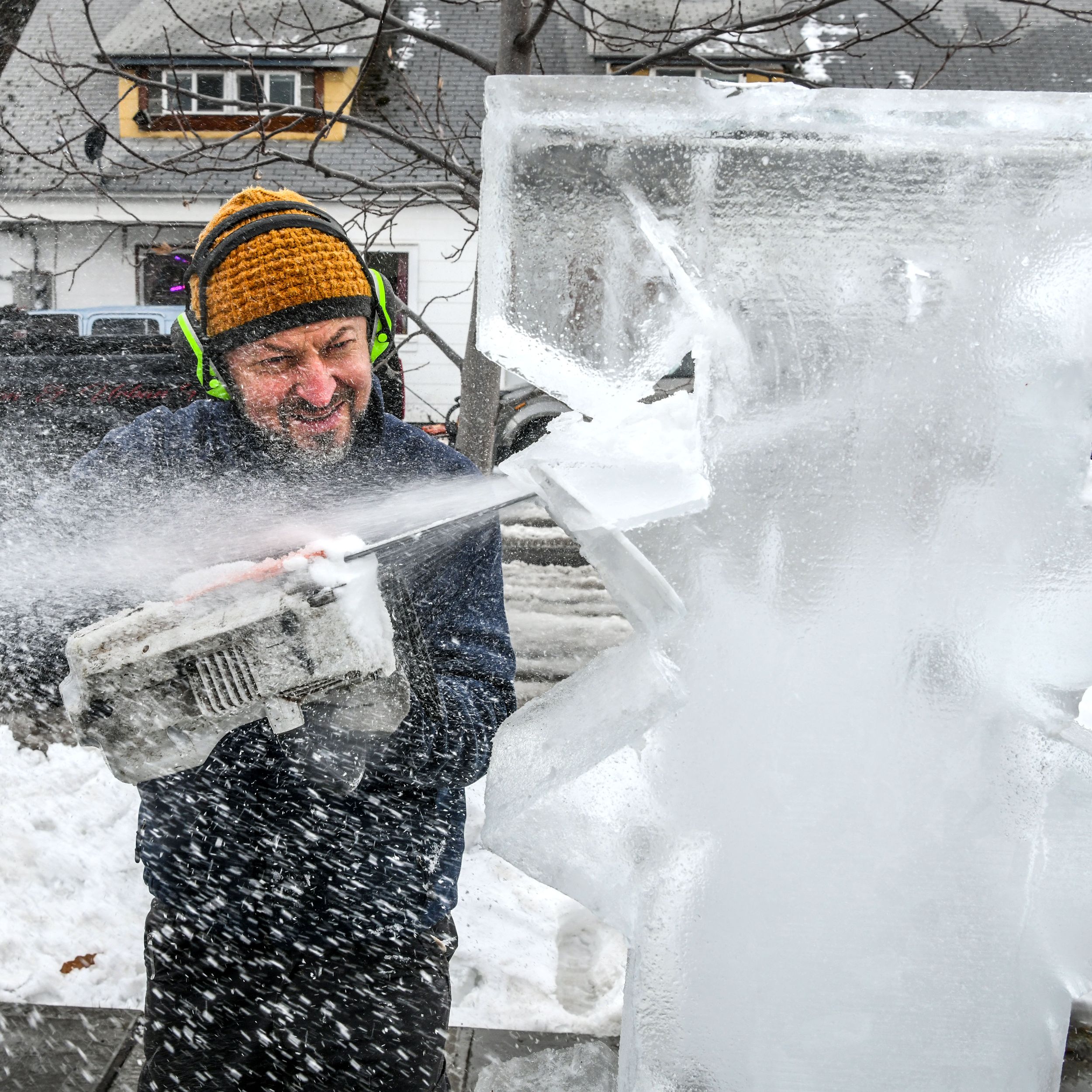The image depicts a bearded man with a goatee, wearing a brown knitted cap with a black rim, along with fluorescent green and black earmuffs. He is intently carving a block of ice with a chainsaw, causing particles to fly off the ice like snow, creating a dynamic and brilliant effect. The scene captures the man in mid-action, with his brow furrowed in concentration. The ice block, positioned in the foreground on the right, displays jagged cuts, giving the impression that it is being shaped into a form, possibly resembling the letter "F". In the background, there is a white house with a gray roof, a snowy road, a truck, and hints of cars, suggesting a winter setting. The presence of fluorescent light and the snowy landscape contribute to the overall cold, festive atmosphere, making it likely that the ice sculpture is being created for an event.